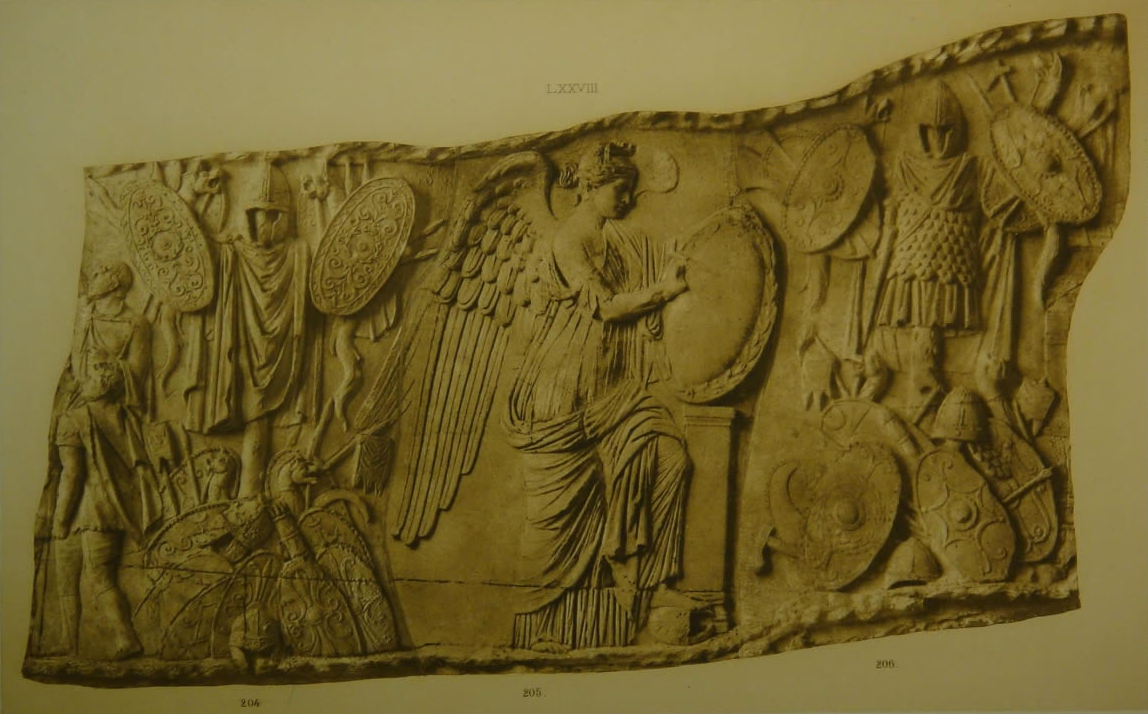The image depicts a detailed, color photograph of an ancient stone relief set against a camel tan background, likely displayed in a museum. The carved stone, with a yellowish-brown hue indicating its age, features an intricate scene that appears to tell a vertical story. On the left, there is a warrior clad in knight's armor, holding two shields, with additional shields at his feet. In the middle, an angel with large wings is depicted in profile, wearing a flowing, loose gown with numerous folds. She holds a round object and has her right foot resting on a rock. To the right, another armored knight is shown, similarly equipped with shields and armor, with multiple shields scattered at his feet. The relief's detailed craftsmanship and the presence of dates at the bottom suggest a historical narrative etched thousands of years ago.